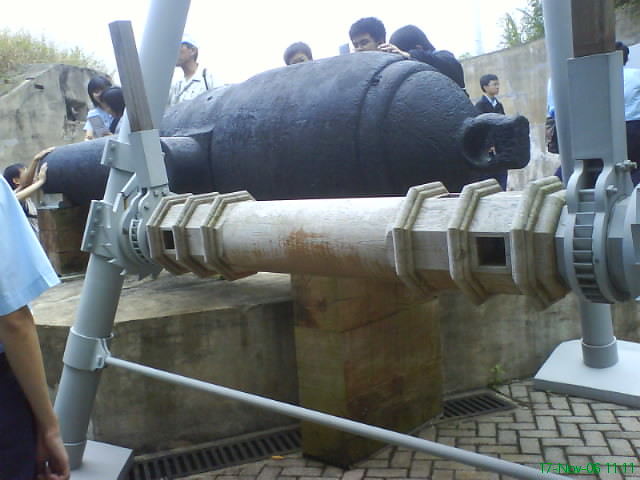The image captures a group of approximately nine individuals, some appearing to be students and others older, surrounding a large, black metallic object that is likely made of steel or copper. The object, which is lying on its side, resembles an ancient bell due to its size, structure, and a distinct hoop at its top. The scene suggests a historical restoration or renovation, set outdoors on a concrete platform, enclosed by concrete walls. The group seems to be engaged in examining, rolling, or pushing the object, possibly loading it using a white metal scaffolding system equipped with levers, gears, and a winch. The scaffolding, with its A-frame design, stands beside what appears to be a decorative, Asian-styled concrete pillar. The individuals, all of Asian descent, are actively interacting with the equipment, some wearing baseball caps, indicating a blend of preservation and educational activity in what could be a museum or historical site.